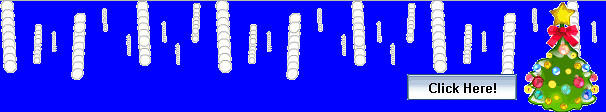A vibrant, royal blue rectangular banner, likely a computer-generated graphic and resembling an internet ad from the early 90s, spans the image. The background is adorned with numerous horizontal white lines resembling segmented rods or caterpillars without faces, varying in size and dispersed randomly from the top to the halfway mark. Towards the bottom-right, there's a festive, green-illustrated Christmas tree decorated in vivid colors: yellow, pink, blue, and red ornaments, topped with a radiant yellow star and a red bow. Adjacent to the tree, a small white rectangle prominently displays the text "CLICK HERE!" in black letters, accompanied by a mouse arrow, further adding to the nostalgic, simplistic digital aesthetic of the graphic.